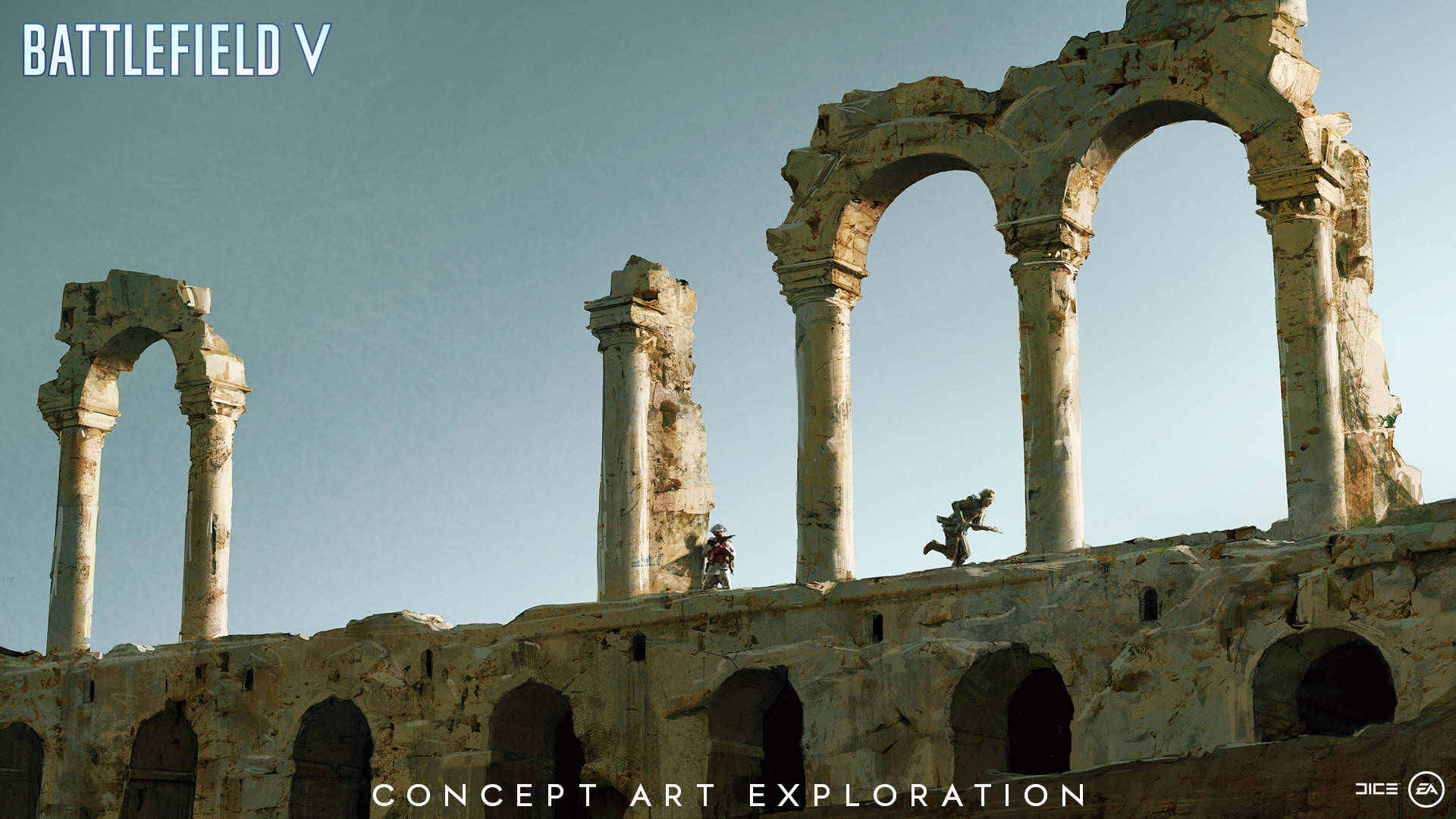This detailed concept art for the video game Battlefield V, created by DICE and published by EA, showcases a battlefield scene set among ancient Roman Greek ruins. The artwork features muted, earthy tones of beige and grey, with sunlight streaming in from the right and casting shadows over the structures. Dominating the scene, an aqueduct and several columns appear partially destroyed and weathered by time, adding an authentic touch to the environment.

Two soldiers are prominently depicted: one is seen dashing forward with a weapon in hand, while the other takes cover behind a column, ready to engage an unseen enemy. The soldiers are dressed in combat gear, complete with hats and weapons, emphasizing the sense of urgency and imminent conflict. The background, painted in shades of blue and grey, hints at an outdoor setting under a brooding sky.

The top left corner of the image is marked by the text "BATTLEFIELD V," while the bottom text reads "Concept Art Exploration," with "DICE EA" also noted, clearly identifying its purpose and creators. The meticulous detailing and atmospheric elements convey the intensity and immersive nature of the game world envisioned in this concept.